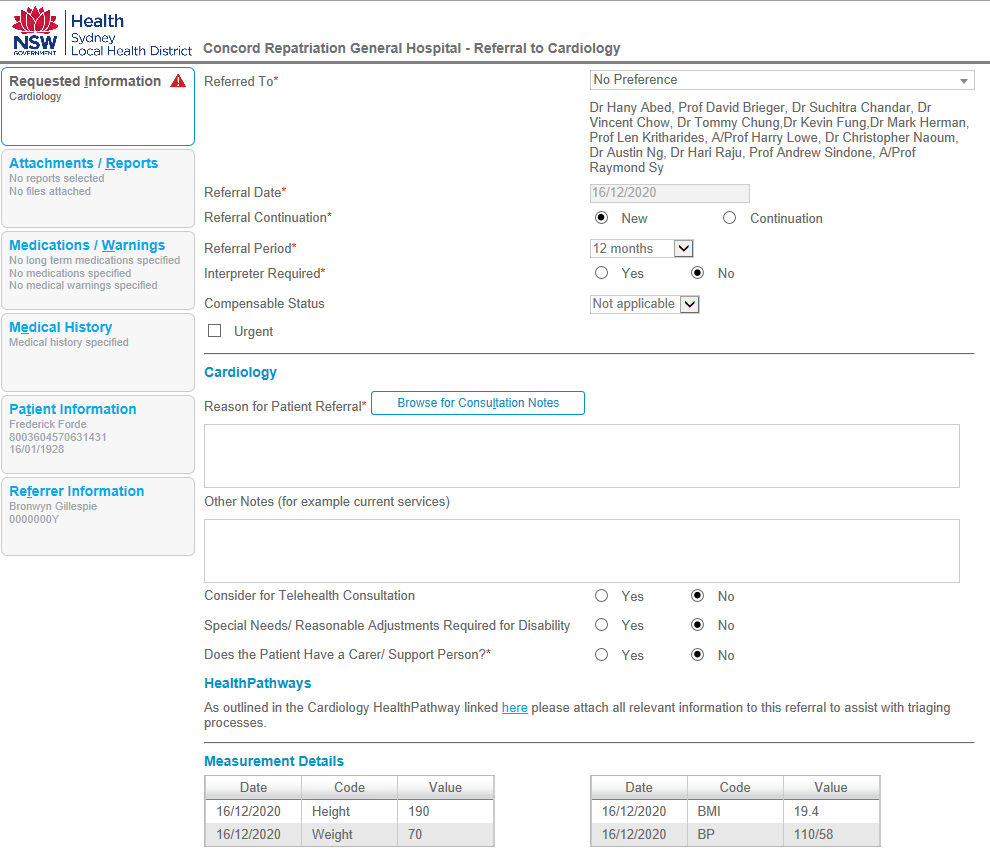Here is a cleaned-up and detailed caption based on the provided description:

---

### Detailed Medical Information Interface from NSW Health

This screenshot shows a comprehensive medical information interface used by NSW Health in Sydney, associated with the Concord Repatriation General Hospital for a cardiology referral. 

**Left Sidebar:**
The left side menu includes:
- Requested Information
- Attachments and Reports
- Medications and Warnings
- Medical History
- Patient Information
- Refer Information

**Main Interface (Right Side):**
- **Referral Details Section:**
  - A section headed by "Referred to" marked with a red asterisk, indicating it's a required field.
  - Below this, fields include:
    - Referral Date
    - Referral Consultation
    - Referral Period
    - Interpreter Required
    - Compensable Status
    - An "Urgent" checkbox

  - A dropdown menu labeled "No Preference" for selecting specific doctors from a long list.
  - A checkbox titled "New" that is already ticked.
  - Additional fields reading "12 months" and "Not Applicable."

- **Cardiology Referral Section:**
  - Headed with "Cardiology" and includes:
    - "Reason for Patient Referral" with an empty white text box.
    - "Other Notes," another white text box.
    - Telehealth Consultation option marked "No".
    - Special Needs and Reasonable Adjustments Required for Disability marked "No".
    - Support Person requirement marked "No".
    - Health Pathways section detailing "as outlined in cardiology health pathway" with a note to attach all relevant information for the triaging process. 

- **Measurement Details Section:**
  - Two data tables labeled "Measurement Details":
    - First table with:
      - Date: 12-16-2020
      - Height: 190 cm
      - Weight: 70 kg
    - Second table with:
      - BMI on the same date: 19.4
      - Blood Pressure: 110/58

This interface encapsulates a detailed and organized methodology for managing patient referrals and medical data in a structured manner.